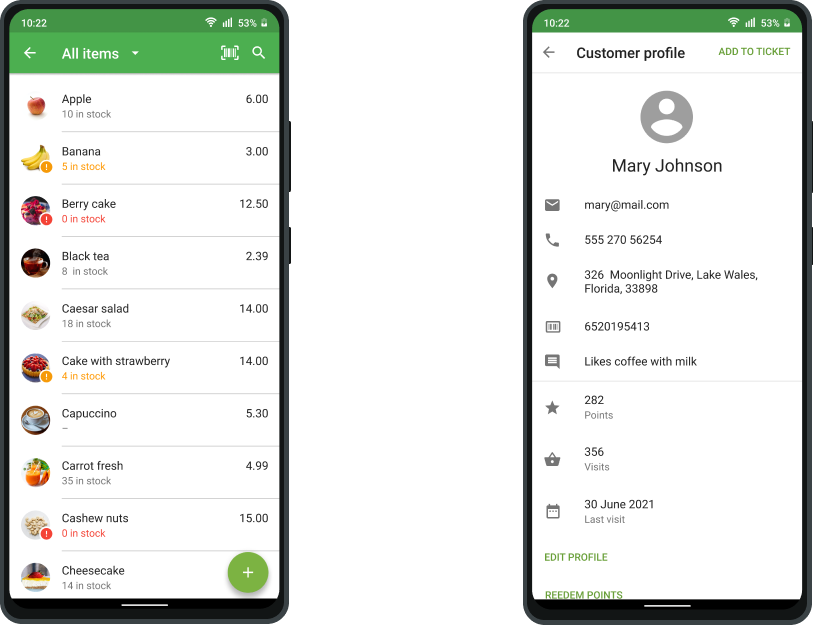Two screenshots of a smartphone are displayed side-by-side, each showcasing a different screen. Both phones have long rectangular shapes with black borders surrounding the screens. At the top of each screen, a small green bar reveals the time as 10:22, with full internet connectivity and a battery level of 53%.

The left screen features a grocery list with 10 items. The first item is an apple, accompanied by an image of an apple. Below "Apple," it indicates "10 in stock," and to the right, the price is listed as $6.00. The second item is bananas, marked with an orange exclamation point indicating only 5 in stock, priced at $3.00. The third item is berry cake, shown with a red exclamation point indicating it is out of stock, and priced at $12.50. Following this are items including black tea, Caesar salad, cake with strawberry, cappuccino, carrots (fresh), cashew nuts, and cheesecake. At the bottom, there is a green circle with a plus sign indicating the option to add more items.

The right screen displays a customer profile at the top, with an "Add to Ticket" button highlighted in green. Below that is a generic avatar icon representing the person, labeled as Mary Johnson. Her contact information is listed as mary at mail.com, with a phone number starting with 505, and her address on Moonlight Drive in Florida. An account number follows, consisting of several digits. Additional details include her preference for coffee with milk, earned rewards totaling 282 points, a shopping basket icon indicating 356 visits, and a calendar noting her last visit on June 30, 2021.